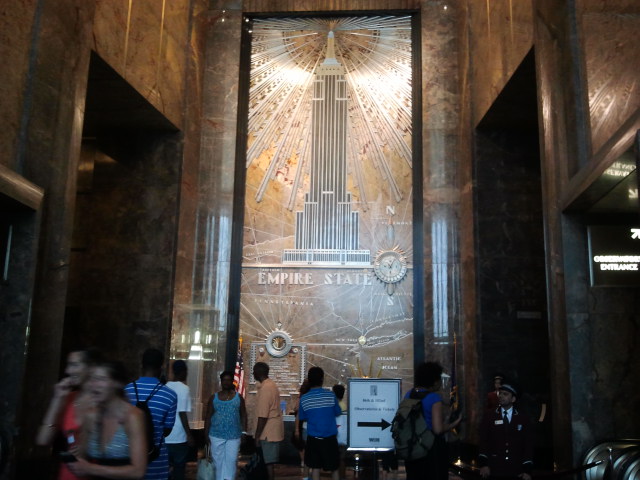The image captures an interior scene of a grand room with towering marble walls and an exceedingly high ceiling that extends beyond what the eye can see. Dominating the center of the room's wall is a large, striking plaque depicting the Empire State Building. Surrounding the building in the image are radiant, sun-like rays that give the structure an almost angelic aura, and below it, in clear bold letters, is the inscription "Empire State." Adjacent to the plaque, there's a functional white sign within a metal frame, featuring a black arrow pointing to the right.

The scene is lively, with numerous people gathered and moving about. To the lower right of the plaque, a security guard stands out in his black uniform, hat, and tie. Nearby, a dark-skinned individual with a backpack and wearing a blue short-sleeved t-shirt is present. Additionally, a dark-haired man dressed in a blue shirt and black shorts looks intently at the Empire State sign. In the bottom left, two women in red and blue tank tops can be seen walking away, adding to the dynamic movement of the scene.